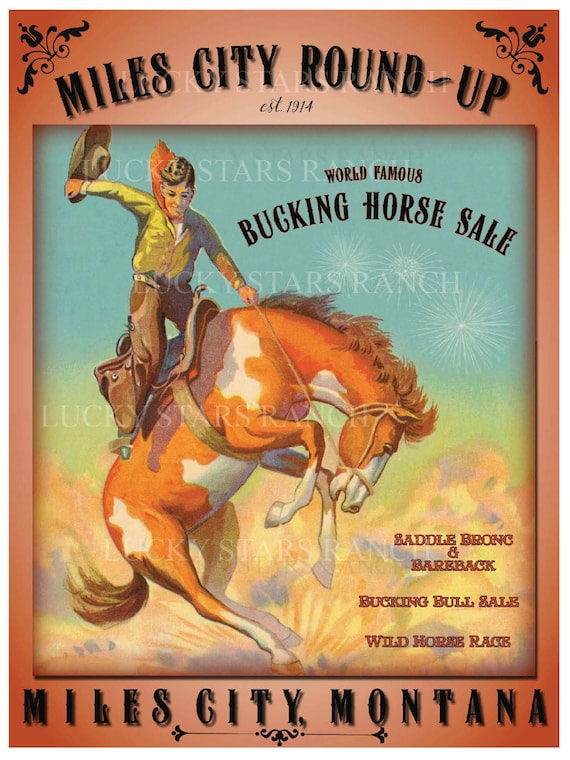This vintage promotional poster, reminiscent of the 1950s era, has a dark pink border with a burnt orange hue. At the top, in bold black letters, it reads "Miles City Roundup, EST. 1914," flanked by small flower designs. The main illustration features a dynamic scene with a young man riding a bucking horse. The rider, dressed in a yellow long-sleeved shirt, a red neck kerchief, and brown pants, grips the reins with his left hand while enthusiastically waving a brown hat in his right. The horse, a striking mix of white and light brown, appears to be mid-buck. Above this action, the words "World Famous Bucking Horse Sale" are prominently displayed. Detailed information at the bottom right of the image indicates "Saddle, Bronc, and Bareback," "Bucking Bull Sale," and "Wild Horse Race." The lower border of the poster is emblazoned with "Miles City, Montana," accompanied by another small flower design, grounding the piece with its geographical significance.